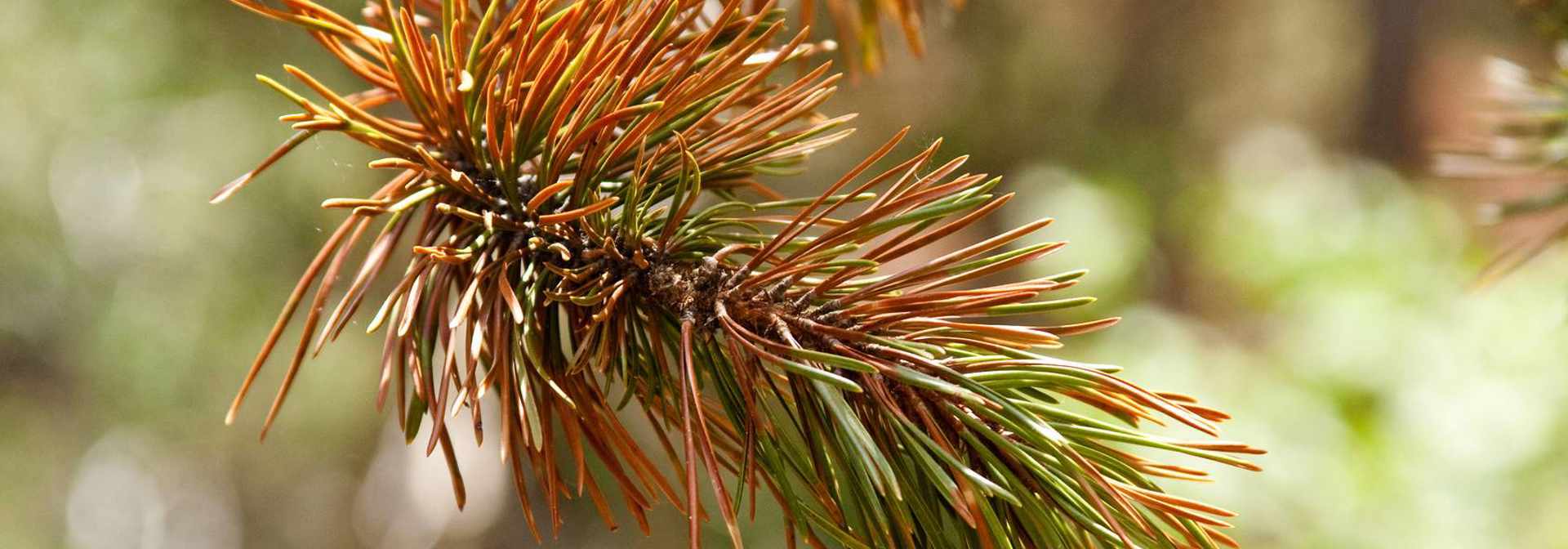This is a highly detailed, macro photograph of a small section of a pine tree branch. The image sharply focuses on the branch, capturing an array of pine needles in various stages of aging. Some of the needles are still vibrant green, while many have turned brown, indicating they are old and possibly ready to fall off with the seasonal change. The branch itself is slightly brown and is positioned prominently in the center of the image. The surrounding background is a blurred mix of greens, suggesting other foliage or trees, but it remains out of focus to draw the viewer's full attention to the intricate details and textures of the pine needles. The sunlight shines softly on the branch, emphasizing the natural hues and the delicate fibers of the needles.